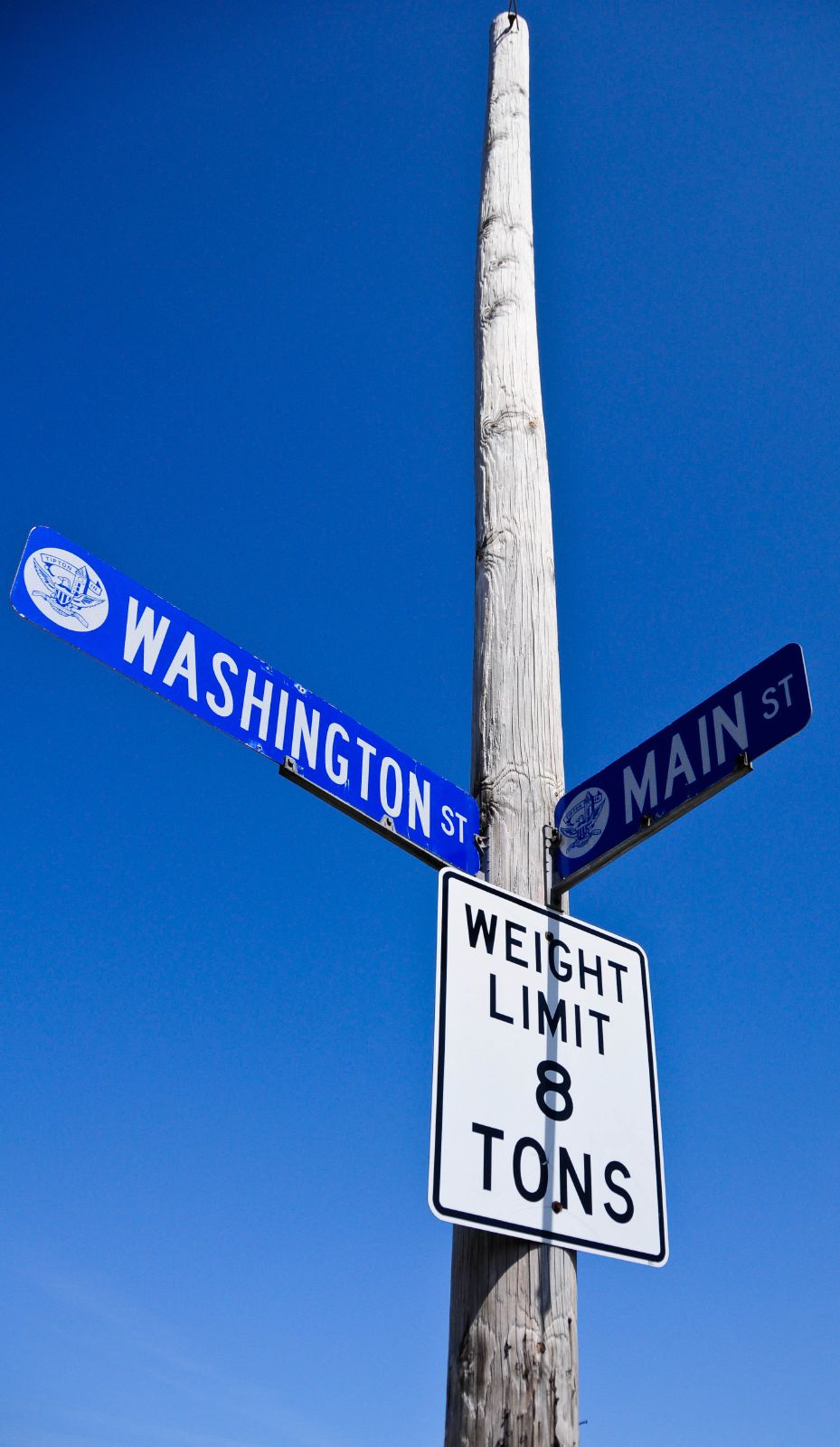Under a gradient sky that transitions from a medium dark blue at the horizon to a deeper, darker blue at the top, a wooden pole stands prominently. Affixed to the pole is a white, square-shaped sign with black letters that indicates a weight limit of 8 tons. Below this sign, two rectangular blue street signs are mounted. The sign on the left reads "Washington St" and the one on the right reads "Main St." Each street sign includes a circular icon, although from the distant perspective of the image, the details within the circles are not clear but they resemble animal silhouettes. The composition captures a serene evening setting with a clear sky and informational signs pointing towards an intersection.